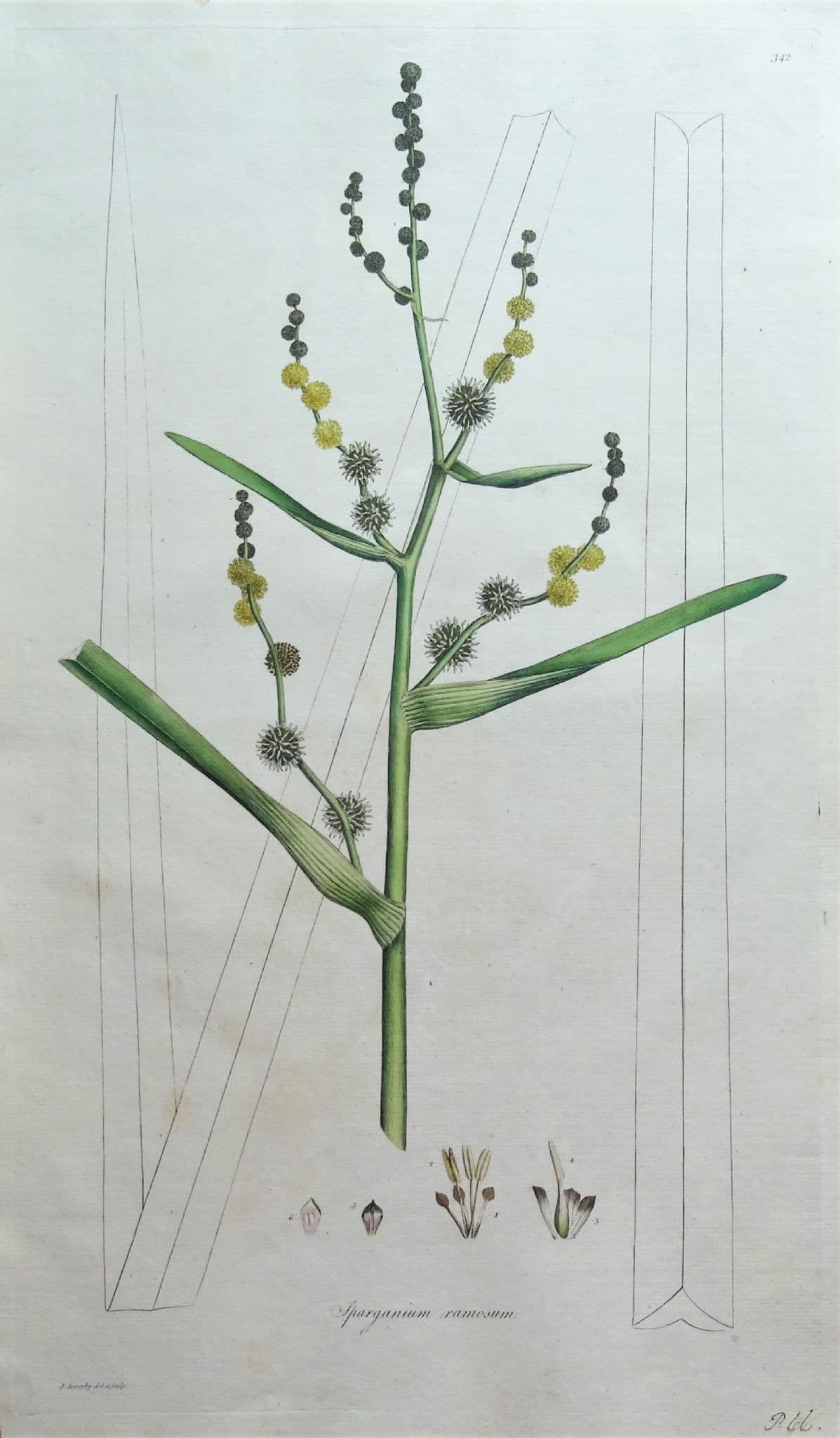This detailed botanical illustration, set against a slightly wrinkled light green background, showcases a unique, tree-like plant featuring a central long, thin stem with narrow, corn stalk-like green leaves. Emerging from the stem are several branches, each adorned with an array of small, globe-shaped blooms. The flowers vary in color, from soft cream to yellow puffs, and include spiky gray to black seed balls and unopened darker gray-green buds toward the branch tips. The image also has pencil or pen outlines of vertical stems or grass blades. At the bottom of the illustration, there are close-up details depicting seeds and other plant characteristics, along with some fine text, likely the scientific name of the plant, though it is too small to decipher.